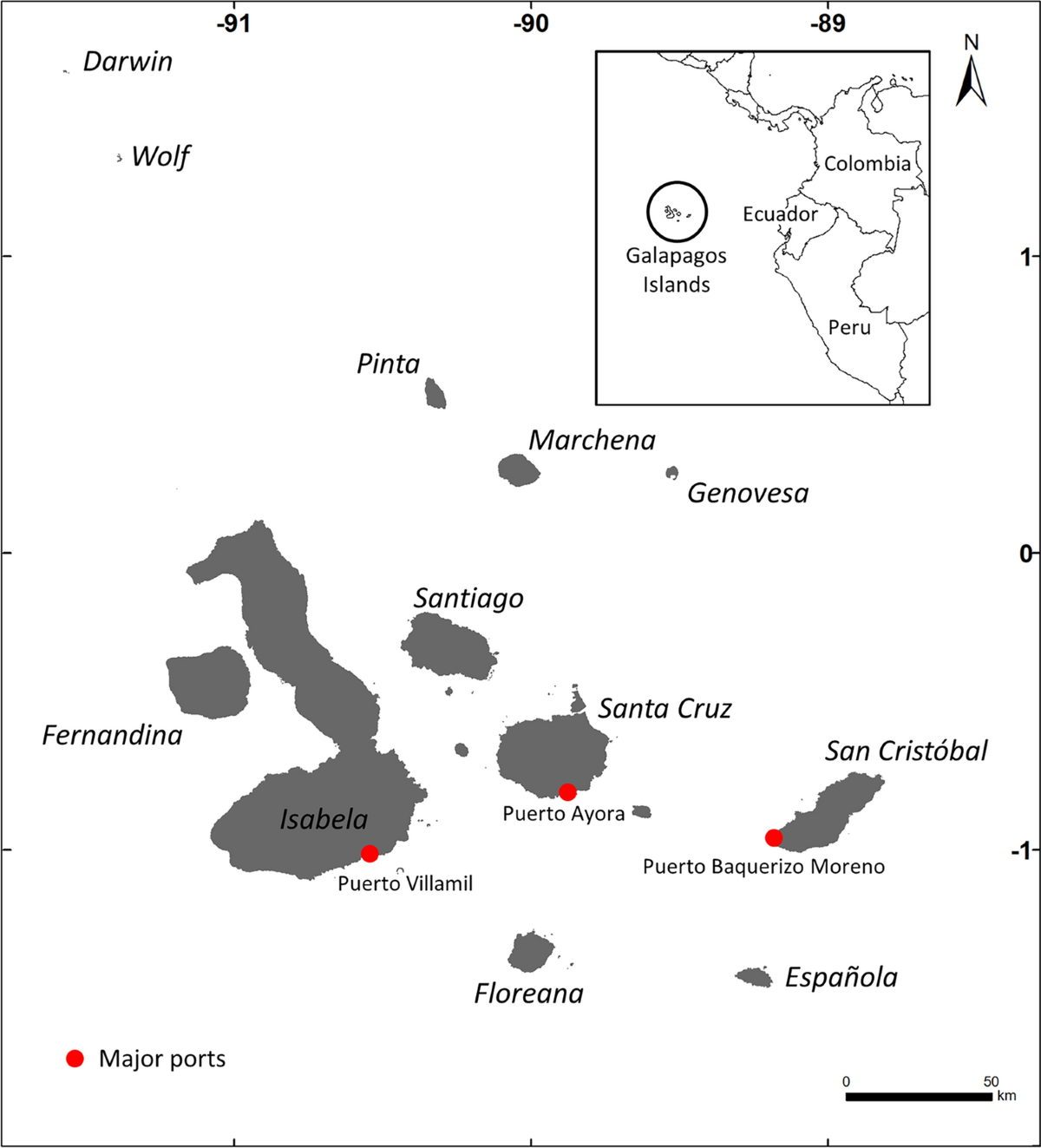This colorful and detailed map highlights the Galapagos Islands off the coast of South America, specifically illustrating the regions surrounding Ecuador, Colombia, and Peru. The main focus is on the Galapagos Islands, where key islands such as Darwin, Wolf, Pinta, Murkina, Genovesa, Santiago, Fernandina, Isabela, Santa Cruz, San Cristobal, Puerto Vilamil, Floriana, and Española are clearly labeled. Major ports are marked with red dots, including Puerto Ayora on Santa Cruz, Puerto Baquerizo Moreno on San Cristobal, and Puerto Vilamil on Isabela. An arrow indicates the north, and a scale for distance measurement is also included. The map's legend clarifies these details and the coordinates, 91° and 90° on the left, and -89° on the right, are marked for precise navigation.